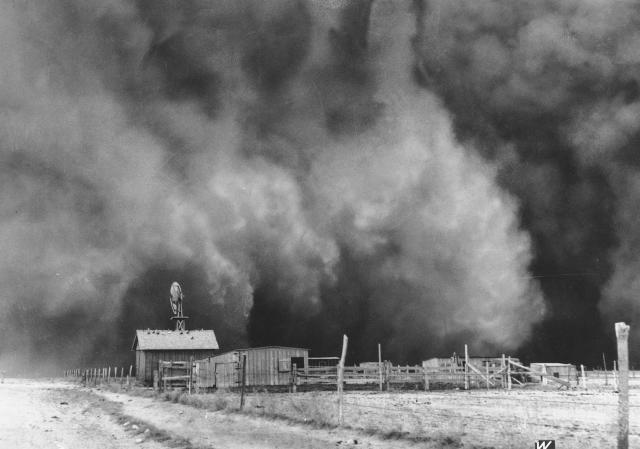This black-and-white photograph captures a barren and desolate farm scene under an ominous sky. The farm, consisting of some dilapidated wooden structures and a rudimentary fence made of widely spaced posts connected by wire, appears vulnerable to the approaching storm. One building stands out with a notably tall structure. The dark road runs parallel to the fence, but the entire landscape is devoid of any human or animal presence, heightening the sense of abandonment. The turbulent gray clouds dominate the majority of the image, encapsulating the small farm community at the bottom in an impending embrace of severe weather. The scene evokes a sense of urgency and foreboding, as if warning of an imminent storm ready to wreak havoc on the already forlorn countryside.